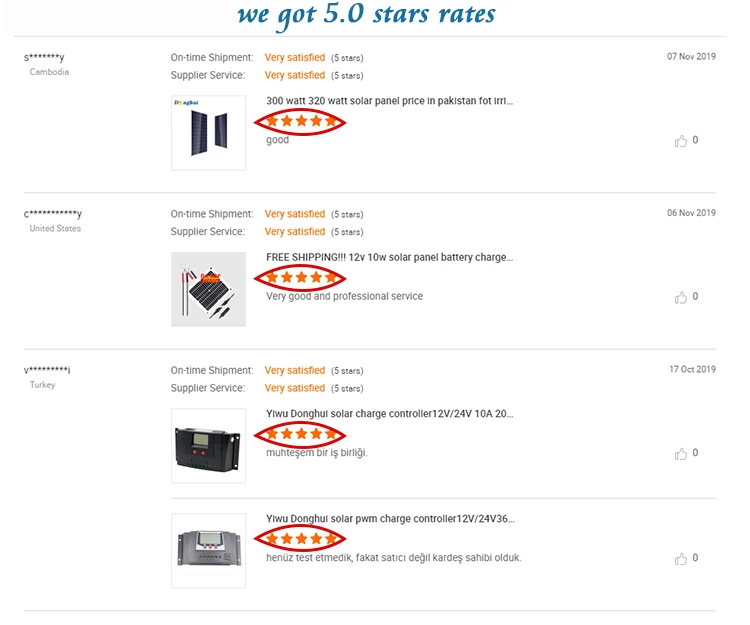A highly detailed image highlights four separate product listings with prominent red circles around their 5-star ratings. The top listing features a black square icon and details a 200-watt to 250-watt solar panel priced from the brand "e-pollet." The second listing emphasizes free shipping and showcases a 12-volt, 110-watt solar panel designed for battery charging. The description also includes a charge controller specification, mentioning "Your thoughts" and a charge controller that supports 12 volts, 24 volts, and 10 amps. The third product is a Ying Droger Solar PWM charge controller compatible with 12-volt, 24-volt, and potentially 36-volt systems. The image concludes with two instances of silence, indicating either blank spaces or undisclosed information.